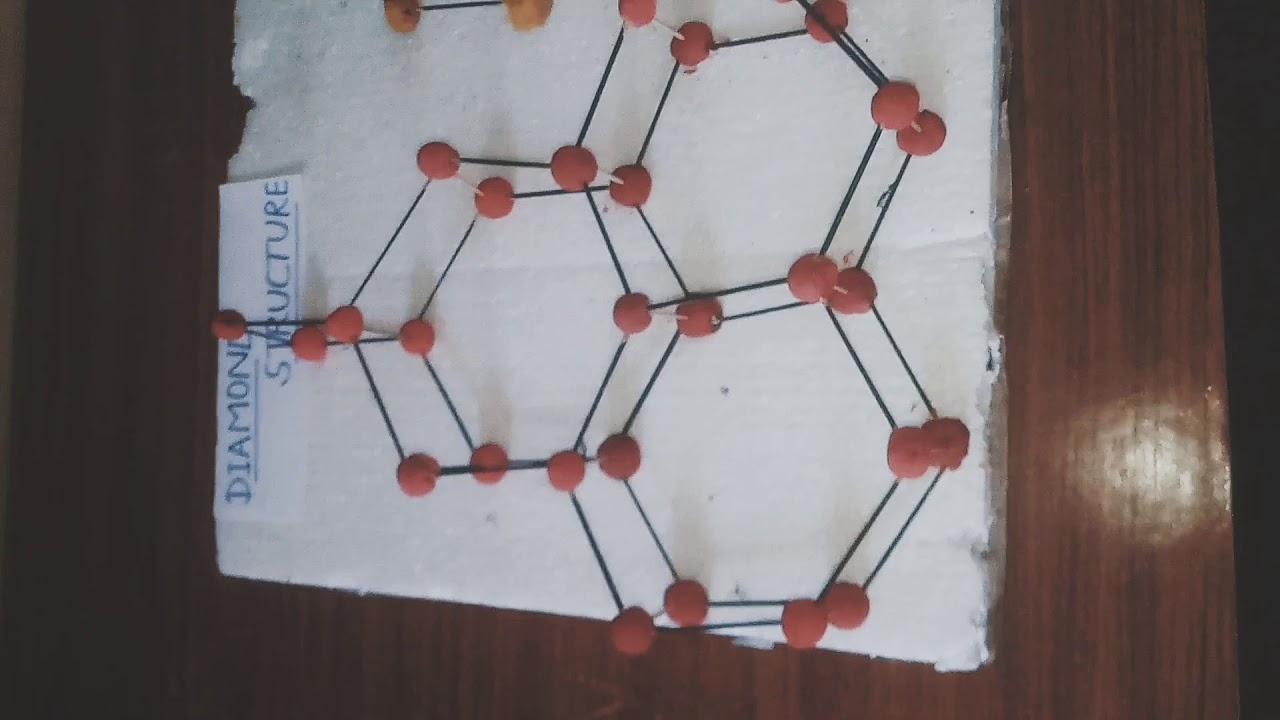The image depicts a detailed 3D model representing a diamond structure, prominently labeled as such in blue, underlined, all-caps text. The model consists of interconnected hexagrams, forming a molecular structure with red balls at each vertex, simulating the atomic components of a diamond. This intricate configuration extends vertically and horizontally, showcasing a network of hexagonal units. The model is mounted on a white surface, which could be either paper-covered cardboard or styrofoam. This base is placed on a wooden surface, suggesting a setting reminiscent of a science fair project or an educational display.